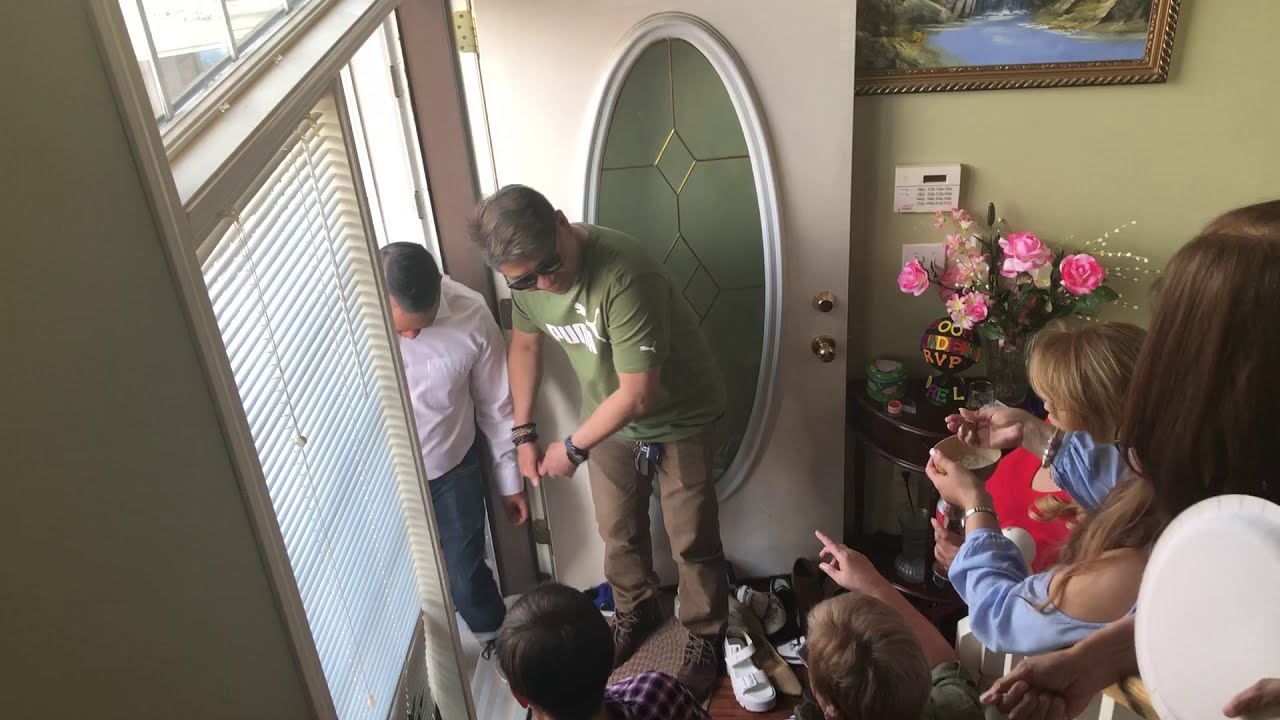In this detailed color photograph, taken from a downward angle as if from a staircase, the scene depicts a family standing in the doorway of a home during what appears to be a midday gathering. The landscape-oriented image features an open front door with an ornate oval beveled glass center, inviting a sense of warmth and welcome. Inside the house, a man in the center wears a dark green t-shirt with a white Puma logo, beige trousers, and sunglasses. Two black and white wrist accessories, possibly watches or bracelets, adorn his wrists as he looks downward. At his feet lies a pile of shoes, indicating guests have recently arrived. 

To the left of this man and slightly outside the door, another individual, dressed in a long-sleeved white top and dark, tight jeans, stands with head bowed, adding to the sense of arrival and transition. Both men serve as focal points for a group of onlookers, primarily children, gathered on the right side of the image. These children, along with the visible back of a woman holding a child, face toward the doorway, indicating curiosity or anticipation. 

The setting's details include a white blind to the left of the doorway, a decorative painting hanging on a green wall in the top right corner, and a table bearing a vase of pink flowers, adding to the domestic atmosphere. The color palette includes tones of white, tan, green, brown, blue, purple, pink, and red, which blend harmoniously to create a welcoming and familial scene captured in photographic representational realism.